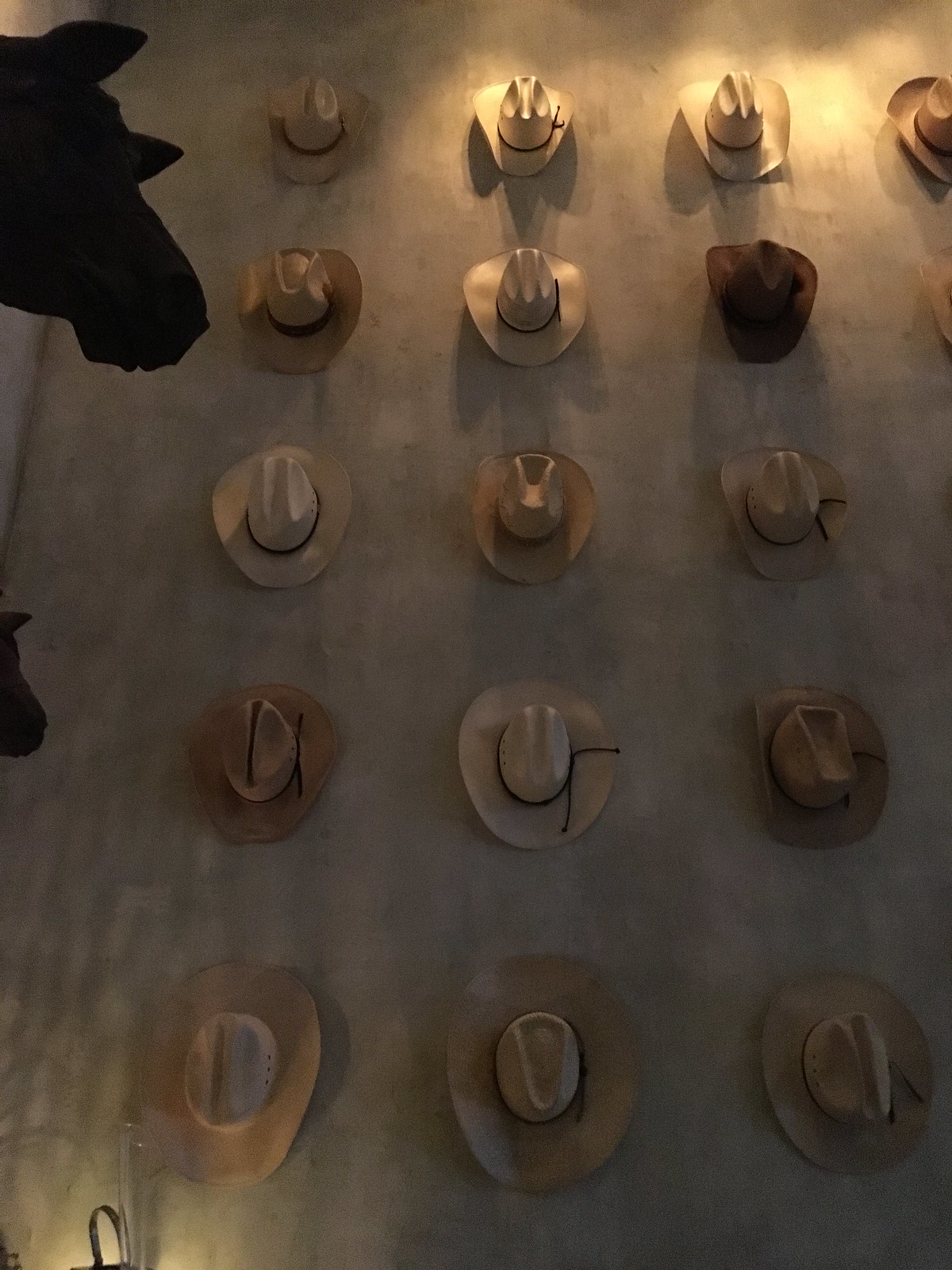This image showcases a striking display of cowboy hats meticulously arranged on a plain, neutral-toned concrete wall. There are five rows of hats, totaling fifteen to sixteen, each with unique characteristics yet sharing a common design feature: a central crease at the top and gently folded brims. The hats vary in color from a near white to a wheat shade, with one notably dark chocolate brown hat standing out. Many of the hats are adorned with bands, adding to their rustic charm. On the wall to the left, the shadows of a horse and a foal—or possibly a moose—add an intriguing element, along with what appears to be part of a purse handle at the bottom. Additionally, a few stuffed creatures are hung up nearby, enhancing the eclectic and visually appealing nature of the scene.